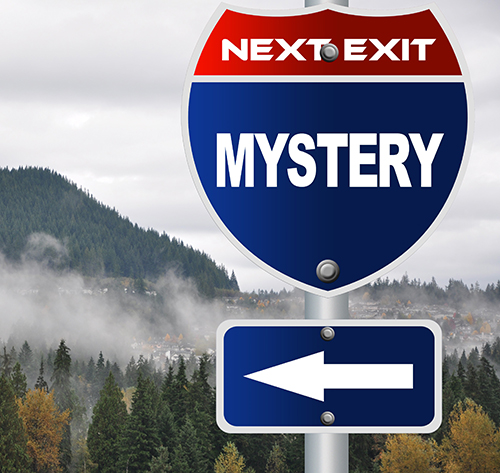This image showcases a digitally-designed sign prominently placed in the foreground against a natural background. The sign, resembling a road sign with a shield shape, prominently displays the words "Next Exit Mystery" in white text. The sign is divided into two color sections: the top third is red, and the remaining two-thirds are blue. Below it, there is a rectangular sign with a white arrow pointing left. The background features an aerial view of an expansive forest dominated by dark green evergreen trees, interspersed with a few yellow or light green trees. The scene extends to reveal a small, partially obscured town, with visible rooftops peeking through a light layer of fog. To the left, a mountain covered in trees rises, all beneath a completely cloudy sky that conceals any hint of blue. This juxtaposition of the vibrant, photoshopped sign with the serene, natural landscape creates a striking and intriguing visual contrast.